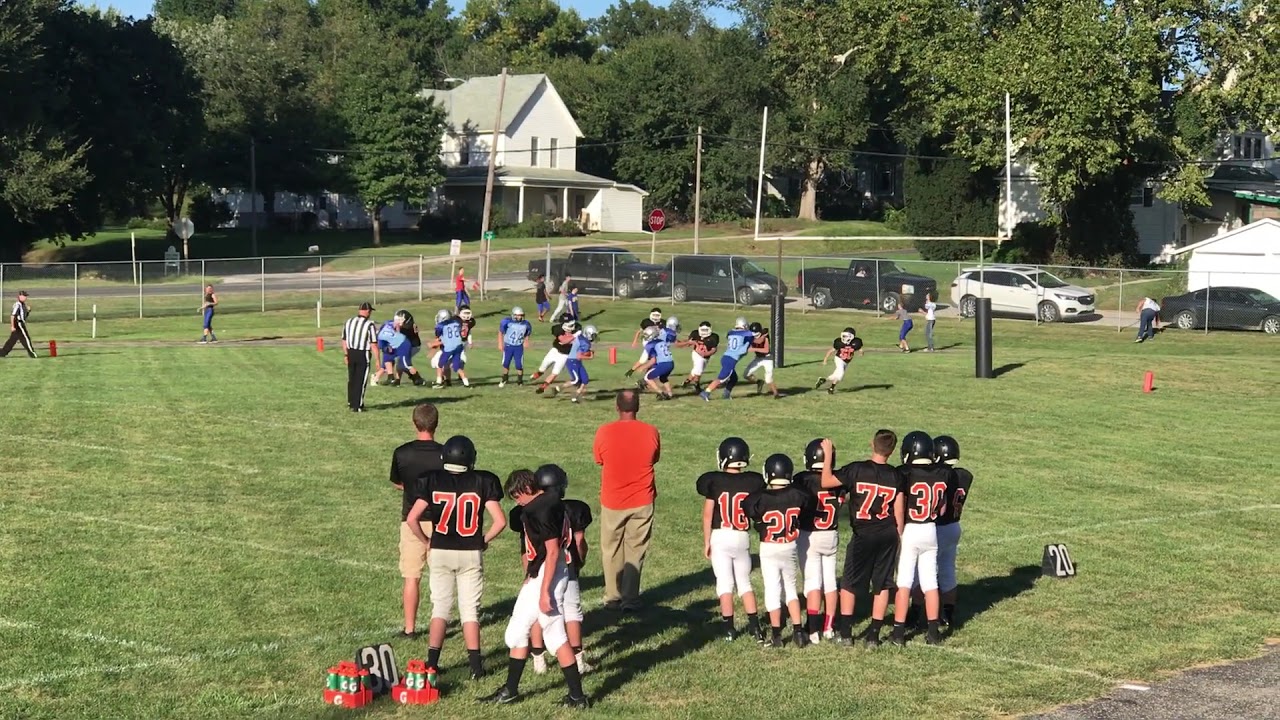In this daytime photograph, we find ourselves on a brightly lit and well-maintained football field. Positioned behind the sidelines, we're situated between the 20- and 30-yard markers. The foreground features a brown-skinned man, balding on top and dressed in a red shirt and khaki pants, engrossed in the game unfolding before him. Surrounding him are young football players, likely middle schoolers around 12 or 13 years old, wearing black jerseys with red numbers, white pants, and black helmets. This team appears to be focused on their teammates who are battling an opposing team outfitted in light blue jerseys and darker blue pants, with silver-colored helmets. 

Scattered on the grass near the 30-yard marker are Gatorade bottles, casting a casual, game-day ambiance. A referee in a traditional black and white striped shirt and cap stands to the left, orchestrating the game. In the distance, another man in a red shirt mirrors our red-shirted man, walking along the far side of the field, accompanied by a second referee. Beyond the chain link fence encircling the field, we see a lineup of parked vehicles, residential homes, and abundant trees, capturing a typical suburban scene on a lively weekend.